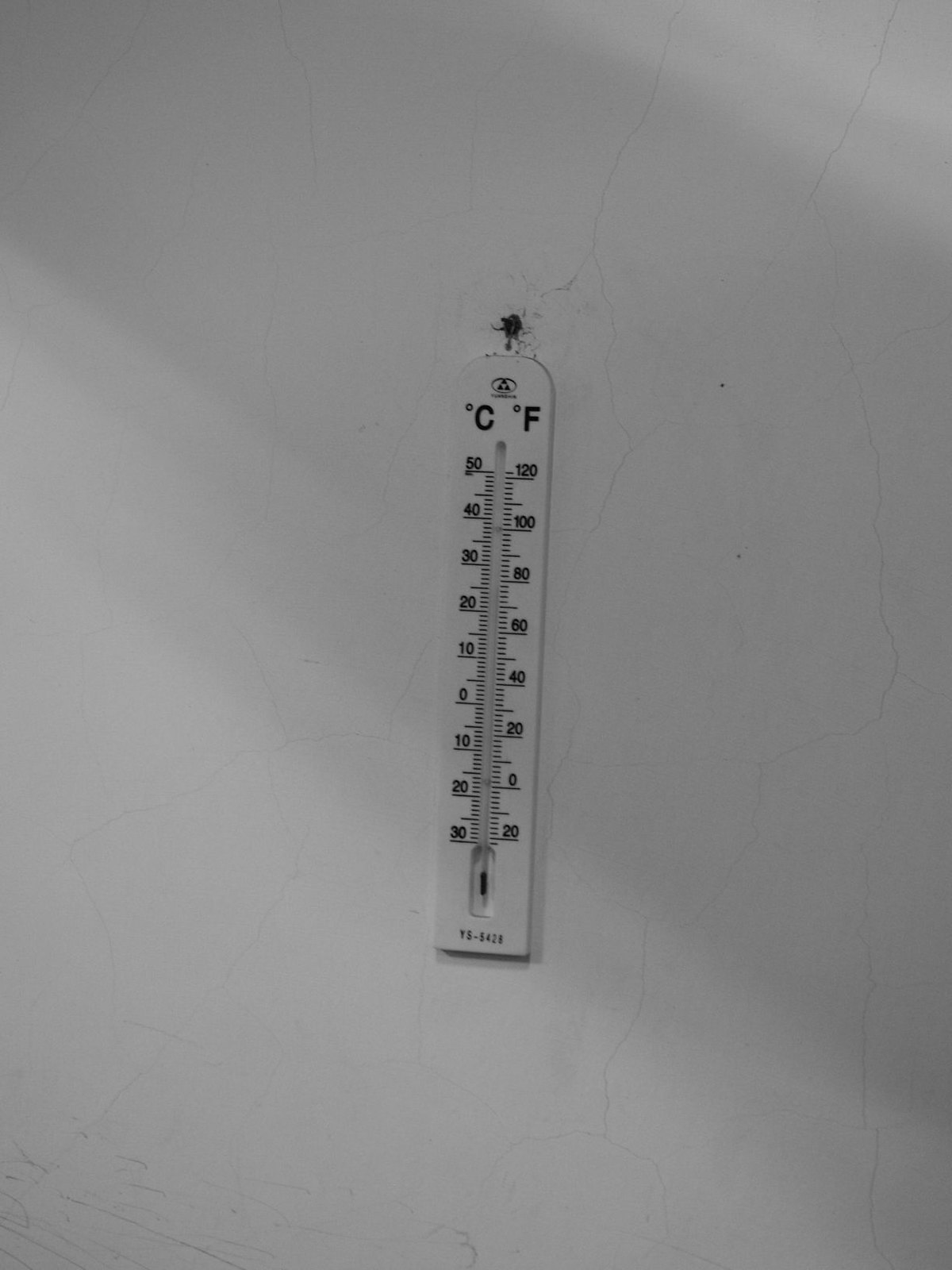The image showcases a wall-mounted thermometer affixed to a white, textured wall with visible lines and vertical cracks extending from the top to the bottom. The thermometer is secured by a nail and features a curved top with a straight bottom. It includes both Celsius (C) and Fahrenheit (F) scales on either side, allowing for temperature readings in both units. Currently, the mercury in the thermometer does not indicate a specific temperature. The background casts a diagonal shadow that spans the entire image, producing a prominent, thick shadow line with two or three narrower lines above and below. The wall appears somewhat dirty, especially around the nail where the thermometer is hung, characterized by noticeable dirt spots. The overall appearance suggests a neglected or well-used environment.